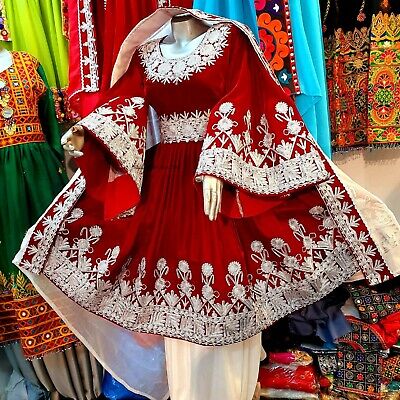The image showcases a vibrant display within what appears to be a fabric or dress shop, filled with colorful and diverse fabrics and dresses. Dominating the center is a striking small red dress adorned with white patterns and intricate designs, prominently mounted on a silver mannequin with visible silver hands and shoulders. The dress is finely crafted with white lace detailing on the neckline, belt, cuffs, and hem, giving it a distinctively elegant appearance, complemented by cream-colored bottoms. Surrounding the central red dress are multiple other dresses and fabrics, including green, orange, blue, and black varieties, some featuring buttons and unique prints like a dragon motif. The assortment of textiles and garments, arranged on mannequins and hanging around the shop, suggests a rich blend of cultural fashion influences, including European and possibly Indian styles, creating a vivid tapestry of colors and textures.